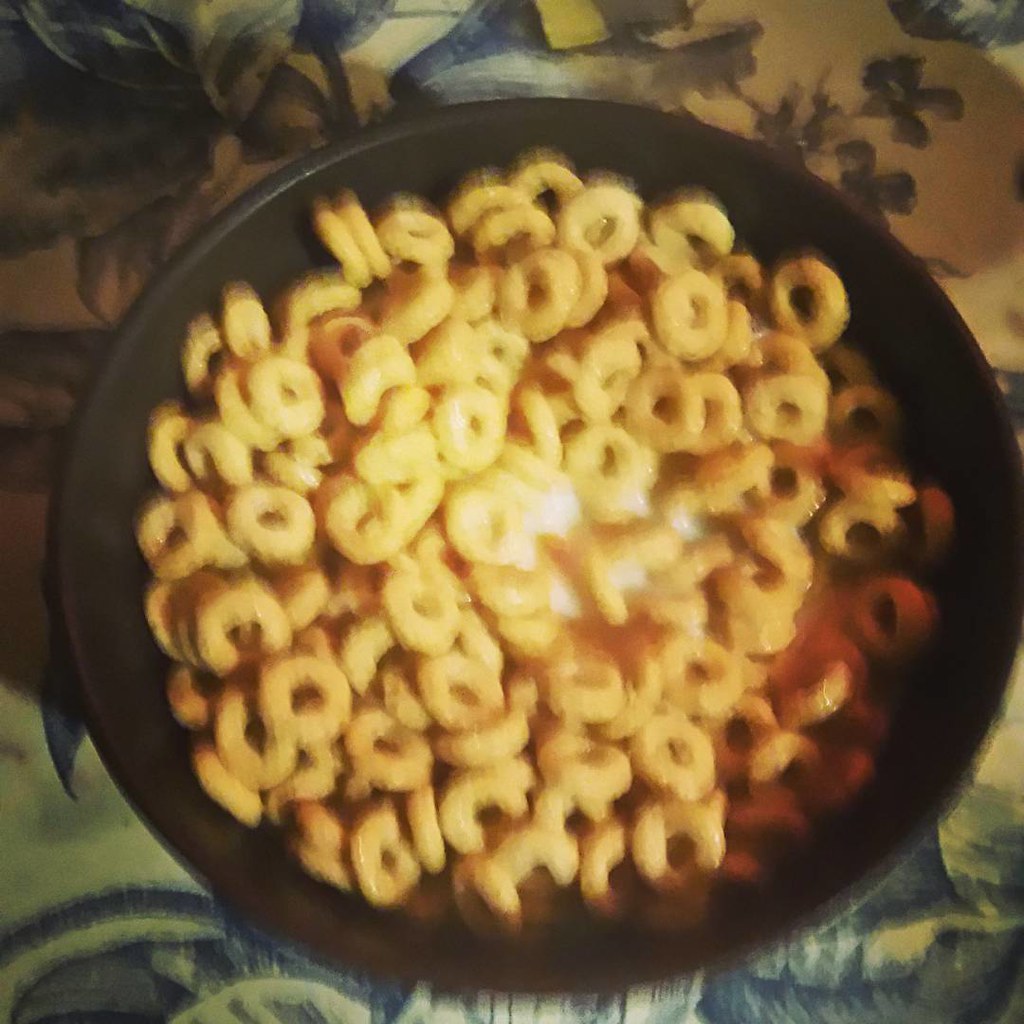This is an overhead photograph of a bowl of Cheerios or Honey Nut Cheerios in milk. The bowl, which is either black, dark green, or possibly brown, sits prominently within the frame, almost touching the edges of the photograph. The cereal consists of yellowish-beige rings, piled above the level of the white milk in the bowl, which is about four-fifths full. Notably, there is no spoon in the bowl.

The background features a detailed, vintage-like floral pattern with blue flowers, leaves, and stems on a yellow or white surface. The exact nature of this surface is unclear, as it could be a tablecloth, a placemat, or even a bedsheet, but it gives a decorative, fancy appearance. The image has a yellowish filter reminiscent of early Instagram photos, contributing to its overall blurry and out-of-focus quality.